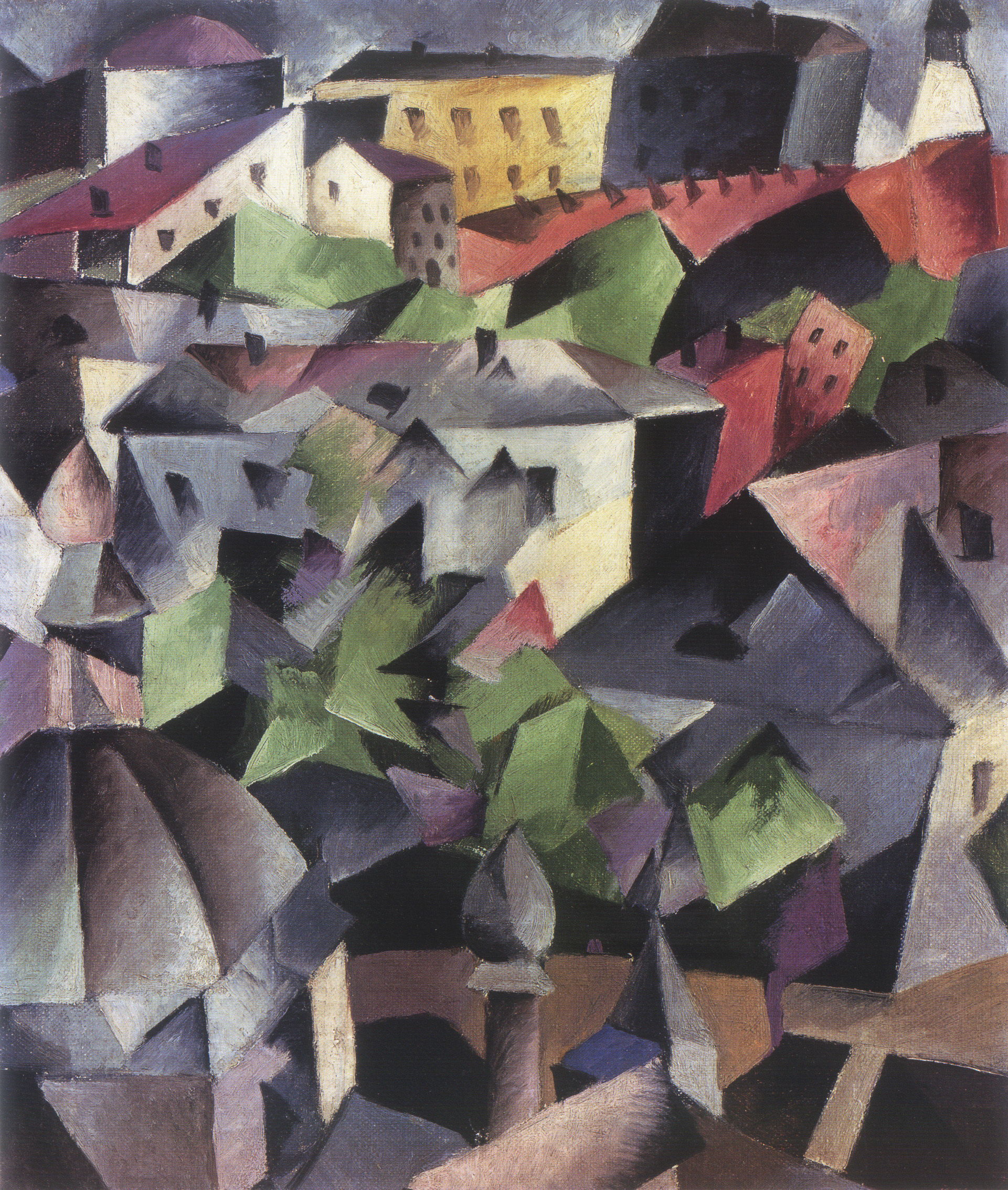The image depicts an abstract, cubist-inspired painting of a city or small village, characterized by straight, geometric shapes that include triangular, square, and rectangular forms. The buildings in the scene are rendered without curves, emphasizing angular and linear design elements. The dominant color palette consists of darkish gray and cream, with several rooftops adorned in red, adding a stark contrast. Interspersed throughout are green blocks, likely representing trees, though they too are depicted in an angular, abstract manner rather than resembling real trees. Distinct from naturalistic scenes, the painting also features details such as small black squares and rectangles to suggest windows and doors, giving form to the buildings. Notably, this painting lacks the presence of people or other objects, focusing solely on the structural elements of the cityscape. The overall style resonates with cubism and abstract art while also incorporating elements reminiscent of modern pop art, evident in the varied color usage and simplistic, almost stylized representations of architecture.